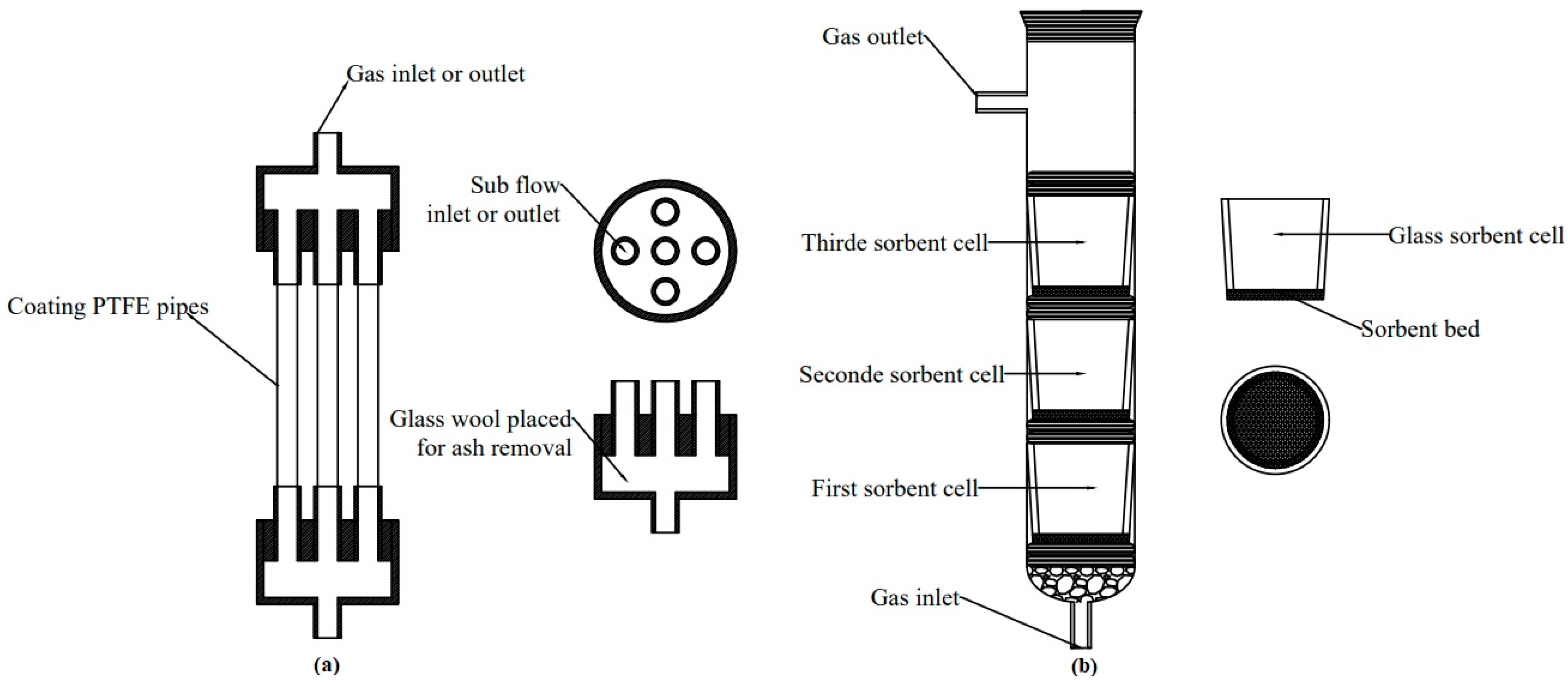This black-and-white diagram illustrates a complex scientific or electrical system involving gas flow through various pipes and cells. On the left side, it features three vertical lines labeled "coding PTFE pipes," which are connected by a top and bottom structure identified as the gas inlet and outlet. There is a circular component marked as the subflow inlet and outlet, along with a section designated for glass wool, specifically placed for ash removal, referred to as Figure A.

Adjacent to this, on the right side, labeled Figure B, there is a taller rectangular structure with multiple designated areas including the gas outlet, a series of disorbent cells (first, second, and third), and other specific labeled sections. This diagram essentially depicts the pathway and mechanisms involved in gas flow from the inlet through various specialized components to the outlet. Each part has its own distinct name and connection lines, making it a detailed schematic of the entire gas system.